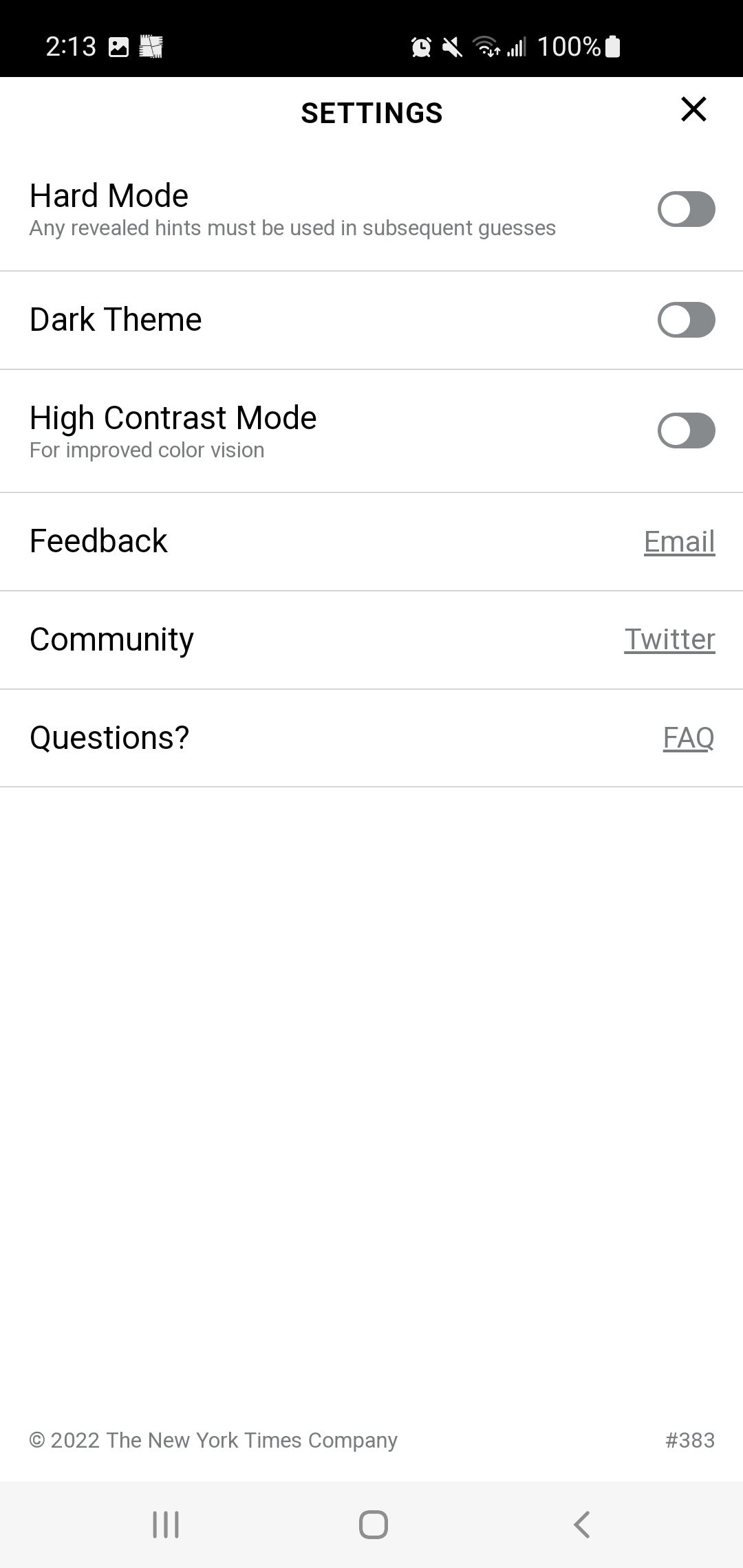This image is a screenshot taken from an Android smartphone, displaying a utility app developed by The New York Times company. The app's interface presents various settings and options. The top section of the screen lists toggles for "Hard Mode," "Dark Theme," and "High Contrast Mode," all of which are currently turned off. Under these toggles, the app specifies that in "Hard Mode," any revealed hints must be used in subsequent guesses. The "High Contrast Mode" is described to improve color vision and is placed beneath the "Dark Theme" option.

Further down, three additional options are presented: "Feedback," "Community," and "Questions." The "Feedback" option allows users to select an email, while the "Community" option links to the app's Twitter page. The "Questions" option directs users to an FAQ section for further assistance.

The app interface is predominantly light-themed, as indicated throughout the design elements. The current time displayed on the screen is 2:13, though it doesn't specify whether it is a.m. or p.m. Overall, the screenshot provides a clear view of the user settings available within this New York Times utility app.